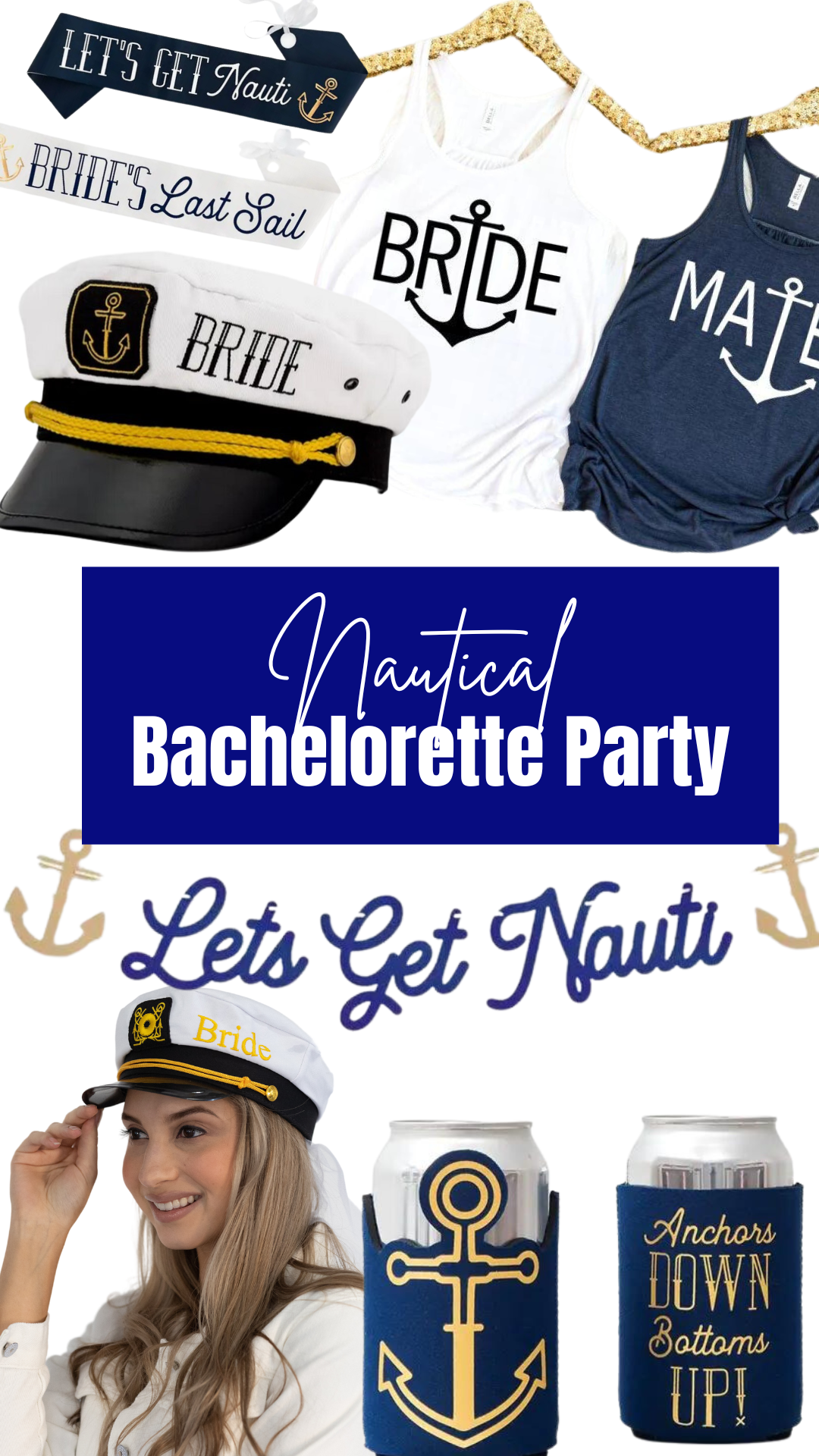The image is a flyer or advertisement for a nautical-themed bachelorette party, featuring various merchandise. At the center, within a blue rectangle, the words "Nautical Bachelorette Party" stand out prominently. Above this, two tank tops are displayed: a white one with "Bride" in black text and a blue one with "Mate" in white text. Accompanying the tank tops is a captain's hat labeled "Bride." 

Additionally, the flyer showcases sashes with playful text such as "Let's Get Naughty," "Nautical," and "Bride's Last Sail." At the bottom of the flyer, two beer koozies with nautical designs and text are featured. In the bottom left corner, a model is seen posing, wearing the bride's captain's hat. The overall design includes nautical elements like anchors and ship themes, all set against a white background to keep the focus on the vibrant and festive party merchandise.